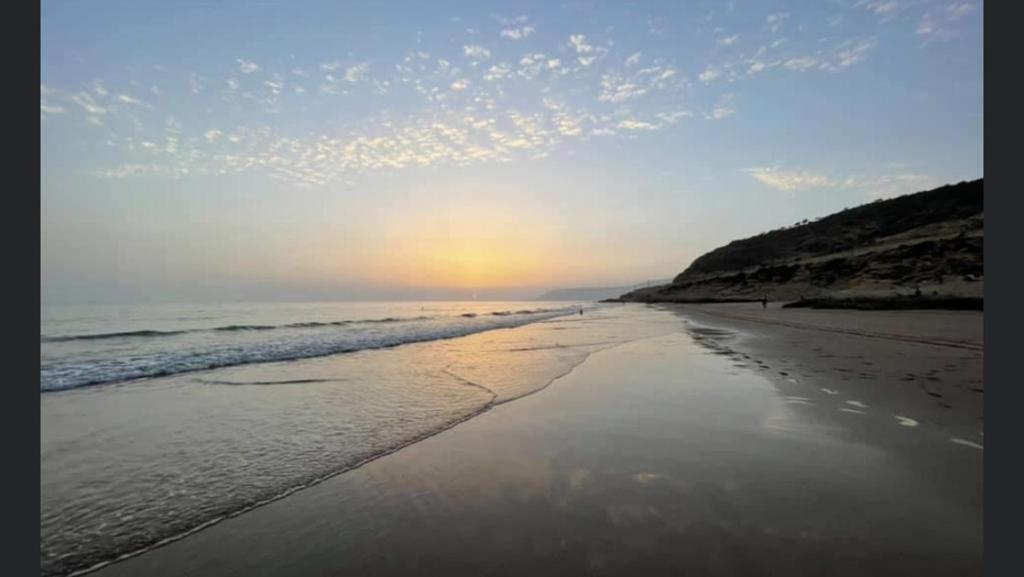The image portrays a picturesque sunset beach scene. Dominating the lower left is the serene blue ocean, where gentle waves break softly onto a wet, reflective sandy beach that stretches across the bottom center and right of the picture. The beach itself is dotted with footprints, adding a sense of activity and human presence. Moving towards the horizon, a dramatic rocky wall, dark and rugged, rises from the right side of the image, enhancing the natural beauty of the landscape.

Above, the sky is split between the warm, glowing hues of the setting sun in the center, casting an orange light across the scene, and the cool blue expanse dotted with speckled white clouds. The sun is poised at the horizon, creating a perfect blend of twilight colors that reflect on the water's surface, creating a mirror-like appearance. In the middle ground, a couple of people can be seen walking, adding life to this tranquil seaside vista. The entire scene is slightly framed by subtle letterboxing on the left and right, focusing the viewer's attention on the breathtaking natural beauty of this beach at sunset.